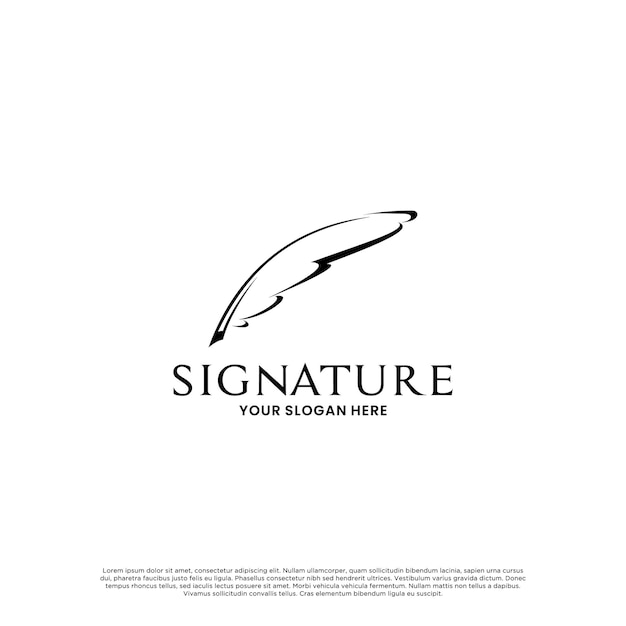This simple and elegant advertisement illustration for a company specializing in business signs features a minimalist design on a white background. At the top of the image is a gracefully flowing, artistic quill pen drawn in black. Positioned centrally in bold, uppercase black letters is the word "SIGNATURE" in a font reminiscent of Times New Roman. Directly beneath it, also in bold black uppercase letters but smaller in size, is the placeholder text "YOUR SLOGAN HERE." At the bottom of the page, there is a block of fine print written in Latin, starting with "Lorem Ipsum Dolar Sit Emet," serving as a placeholder for additional text. The overall design is simple yet visually appealing, making it an effective and customizable advertisement.